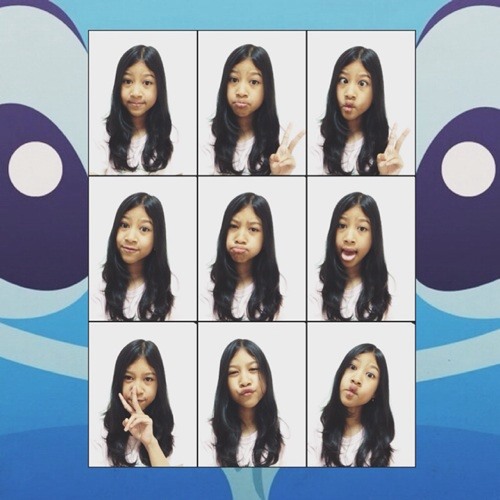This image is a series of nine vertically rectangular headshots of a preteen girl, around 10 to 12 years old, displayed in a 3x3 grid. She has long, straight black hair parted at the center, tan skin, and appears to be of Hispanic or Asian descent. The background for each photo is a plain white, and the entire grid is framed by a blue and purple border that features two split, wide-open eyes, creating a whimsical backdrop with a gradient from light blue to dark blue.

In the top row, starting from the left, the first photo shows the girl with a neutral expression. In the second, she has a pouty face while holding up a peace sign. The third picture features her cross-eyed with puckered fish lips, still giving a peace sign. The middle row begins with another neutral photo, but this time her head is slightly tilted. The middle image shows her with puffed-out cheeks and pouty lips, and the rightmost picture captures her with a wide-open mouth, though the rest of her face remains expressionless. In the bottom row, the left photo again includes a peace sign, which covers part of her face, leaving her expression neutral. The middle photo shows her making a pouty, kissy face with semi-closed eyes, and the final image features her with puckered fish lips and wide-open eyes, her head slightly tilted.

Overall, the series captures the girl's playful and expressive personality, showcasing a variety of goofy faces and fun poses typical of a photo booth session.